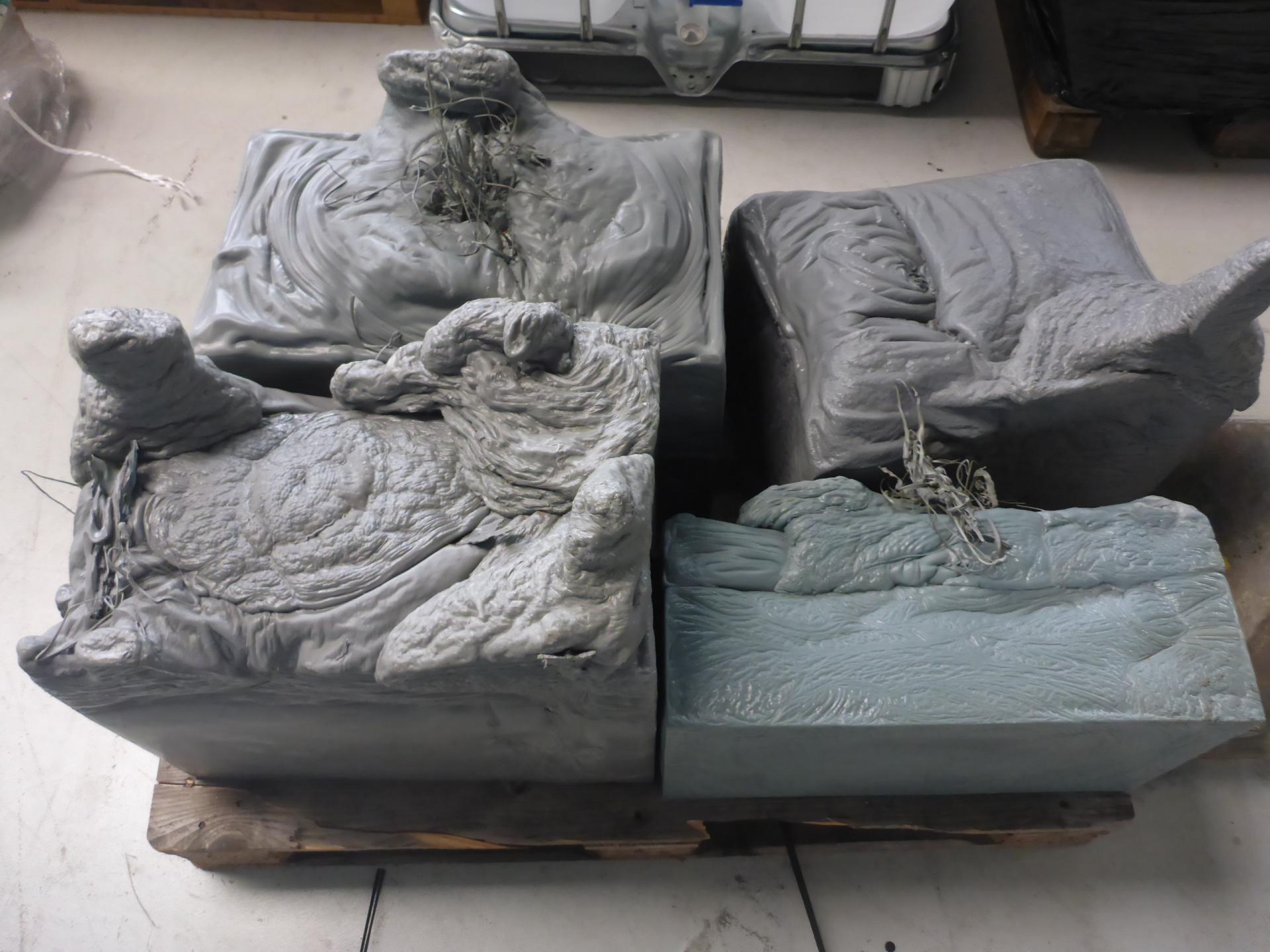The image captures an overhead view of four gray sculptures situated on a wooden slatted platform. These sculptures, which may resemble foam blocks, exhibit various degrees of warping and misshaping at their tops, giving them an almost wet or not fully dried appearance. The platform itself rests on a gray wood-planked floor, distinguished by two black grout lines at the forefront.

The sculptures vary in shape, with one noticeable square piece in the upper right corner leaning to the left, almost pillow-like. The sculpture in the lower left-hand corner is about a foot high, with its corners built up, possibly evoking the shape of a mountainous landscape or a castle. Ropes or strings are visible between some of the objects on the right side, adding an element of texture.

In terms of color, the sculptures range from dark gray to shades that verge on a bluish tint. Additionally, portions of what appear to be furniture—potentially a white chest—are partially visible in the upper right corner of the image, contributing to the ambient setting.